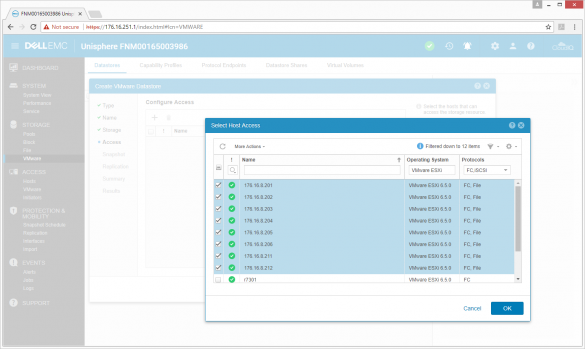This photo captures a web browser window, albeit slightly blurry, with several discernible details. The upper left-hand corner features a tab displaying black font for the title. Despite the blurriness, a long string of numbers is visible within the title. The tab itself is gray, with the web address located underneath and to the right of standard navigation buttons—the back arrow, forward arrow, and refresh button. The web address bar displays an "Not secure" warning alongside a partially visible IP address, starting with "HTTPS" and including "look star 176." In the main viewing area of the browser, the top left-hand corner prominently features the label "Dell EMC," with "Unisphere" noted to the right of it. The central focus of the image is a pop-up window acting as the main interface, which lists several IP addresses each accompanied by checkboxes.